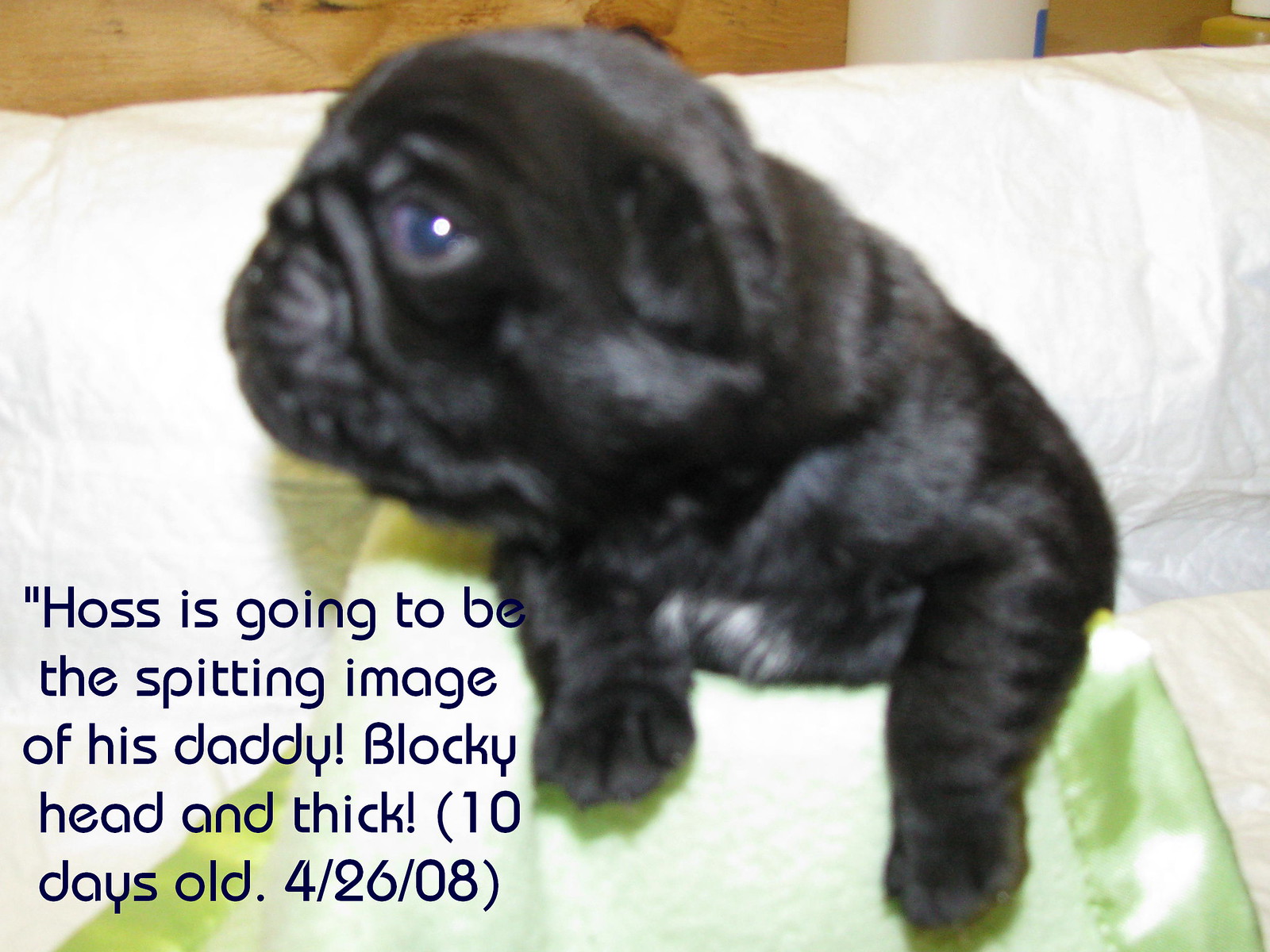This close-up photograph captures an adorable black pug puppy, just 10 days old, resting on a soft surface within a cozy bed. The background features a mix of green and white fabrics, with a hint of a brown object visible as well. The puppy, exhibiting puppy dog eyes that appear somewhat blue, sits partially under a green blanket, almost like a human. His head is slightly tilted, showcasing his cute, wrinkly face and soft, well-groomed fur. Text in black on the bottom left corner of the image reads, "Haas is going to be the spitting image of his daddy. Blocky head and thick. 10 days old. 4/26/08," indicating the potential resemblance to his father. The intimate setting and the loving presentation suggest that this might be a cherished moment shared on social media.